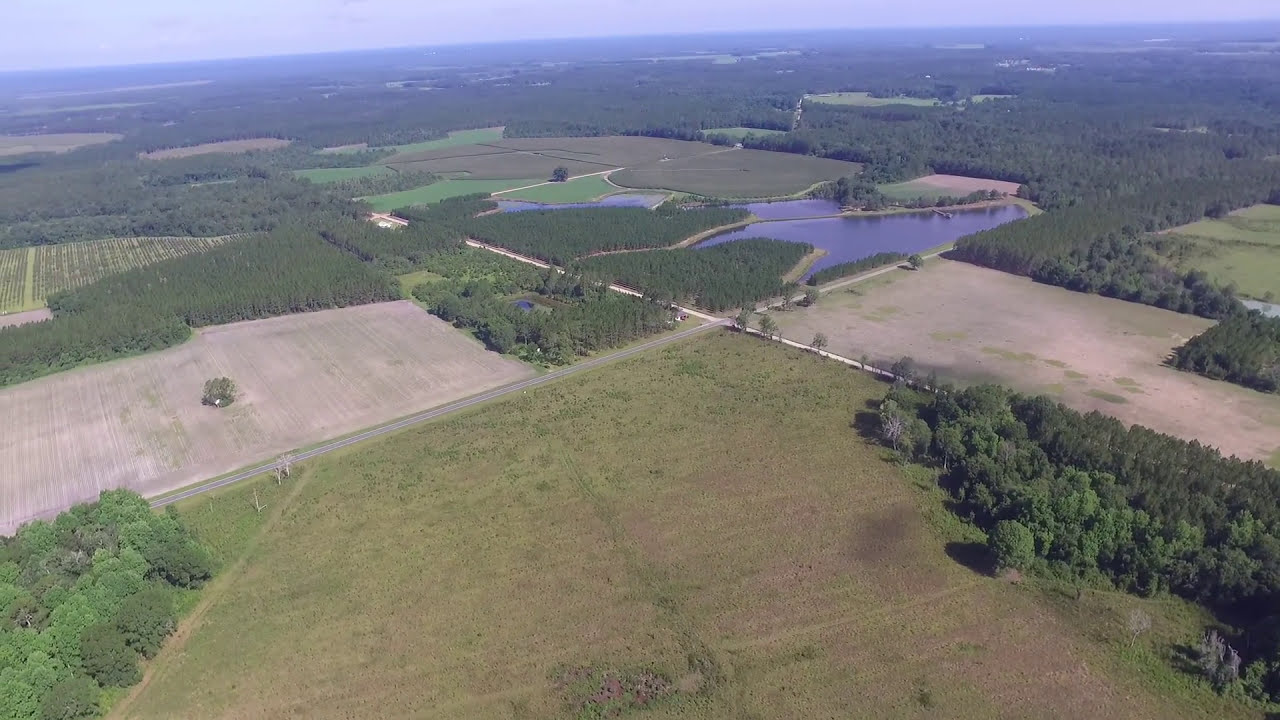This aerial landscape image showcases a serene countryside devoid of buildings. At the bottom center, an open field stretches out, flanked by clusters of lush green trees to the right and left. A long road meanders across the scene, its gray surface marked with white lines, connecting the different areas. Moving further into the image, several smaller bodies of water, including a prominent blue lake, punctuate the expanse of tan and green fields. The fields continue to extend into the distance, interspersed with more green patches and trees of varying shades, creating a patchwork effect. The background gradually blends into a bluish sky, completing this tranquil and picturesque rural setting.